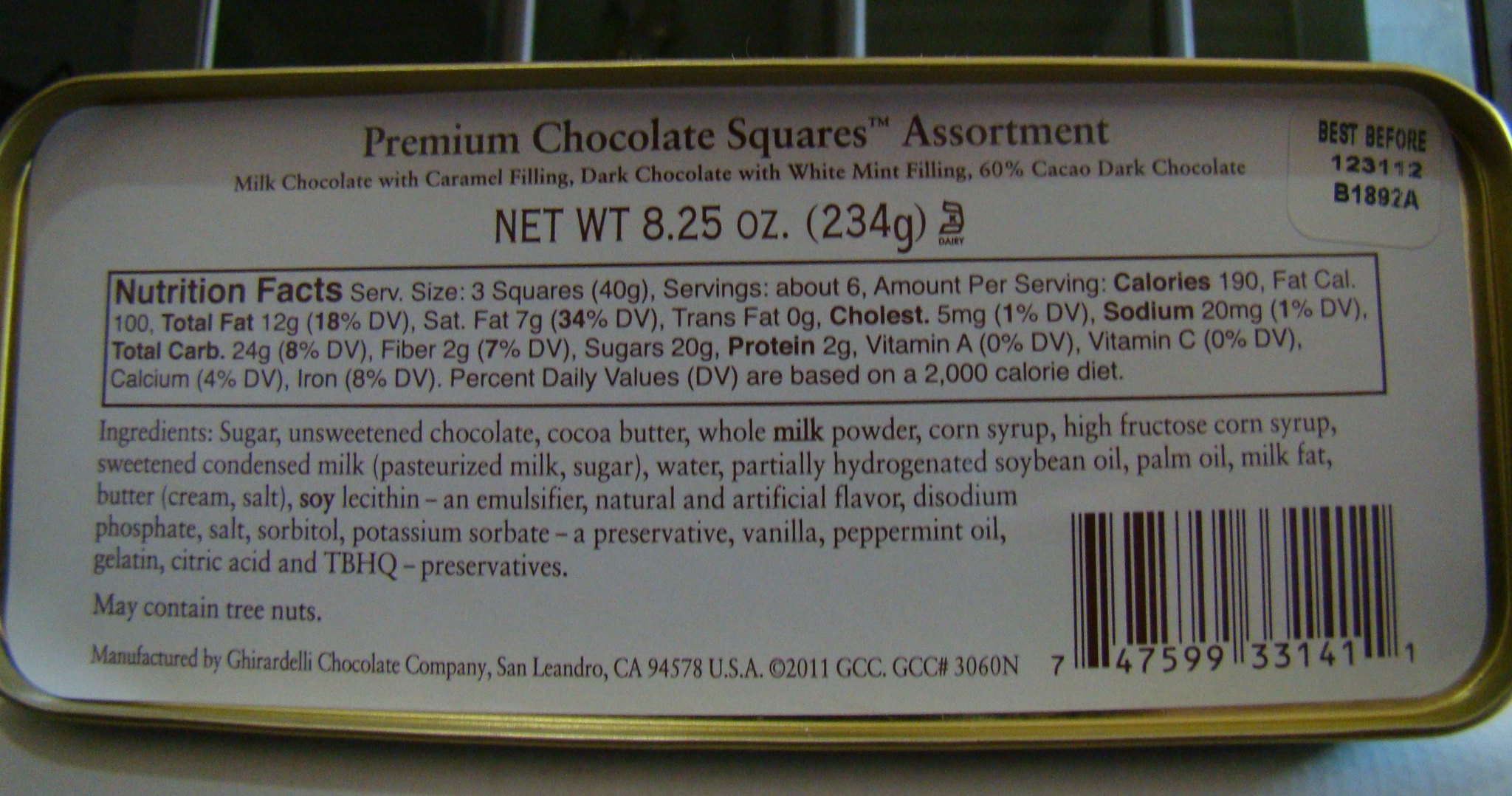This image features the bottom of a tin of assorted premium chocolate squares. The tin includes various flavors such as milk chocolate with caramel filling, dark chocolate with white mint filling, and 60% cocoa dark chocolate. The net weight of the contents is 8.25 ounces (234 grams). 

In the top right corner of the tin, there is a white sticker displaying the best before date marked as "123112B1892A." There is also a detailed list of ingredients, including sugar, unsweetened chocolate, cocoa butter, whole milk powder, corn syrup, high fructose corn syrup, sweetened condensed milk, water, partially hydrogenated soybean oil, palm oil, milk fat, butter, soy lecithin (an emulsifier), natural and artificial flavors, disodium phosphate, salt, sorbitol, potassium sorbate (a preservative), vanilla, peppermint oil, gelatin, citric acid, and TBHQ preservatives. The tin notes a potential for containing tree nuts. 

Additionally, a barcode is present in the bottom right corner of the tin. The overall design and information provided are clear and concise, ensuring the consumer is well-informed about the product's contents and nutritional information.